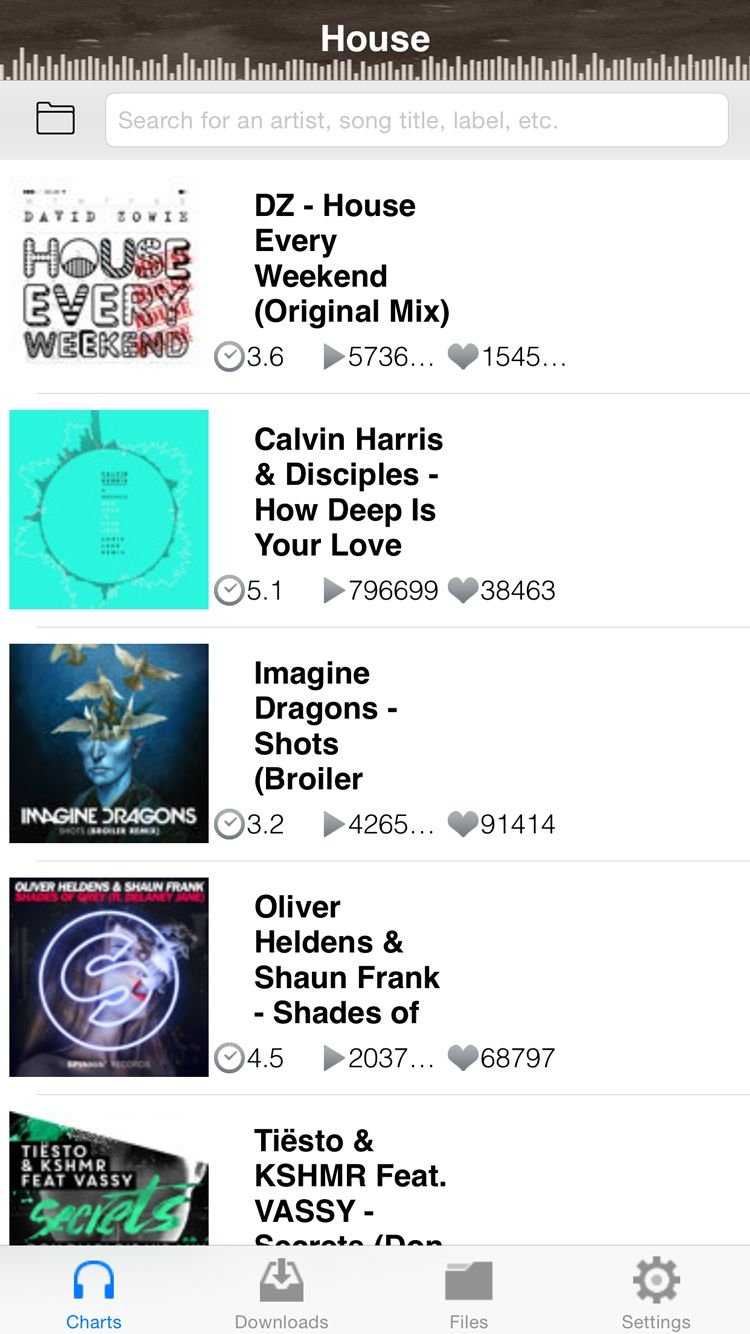**Screenshot of a Music Download Program Interface**

At the top of the web page, the title reads "House" accompanied by several navigation bars. This appears to be a screenshot of a music download program, showcasing various songs available for download.

1. **Song Title: House Every Weekend (Original Mix)**
   - **Rating:** 3.6 stars
   - **Plays:** Approximately 5,736 plays
   - **Likes:** 1,545 likes

2. **Artist: Calvin Harris & Disciples**
   - **Song Title: How Deep is Your Love**
   - **Rating:** 5.1 stars
   - **Plays:** 7,969,699 plays
   - **Likes:** 38,463 likes
   - **Artwork Description:** The artwork resembles a Linnean evolutionary scale.

3. **Artist: Imagine Dragons**
   - **Song Title: Shots**
   - **Rating:** 3.2 stars
   - **Plays:** 4,265 plays
   - **Likes:** 91,414 likes
   - **Artwork Description:** The image features a human head with dragons or birds flying out of it.

4. **Artists: Oliver Heldens & Shaun Frank**
   - **Song Title: Shades of Grey**
   - **Rating:** 4.5 stars
   - **Plays:** 2,337 plays
   - **Likes:** 6,802 likes
   - **Artwork Description:** The artwork displays a large neon "S."

5. **Artist: Tiësto & KSHMR featuring Vassy**
   - **Song Title: Secrets**
   - **Rating:** Information cut off in the screenshot

At the bottom of the interface, the following tabs are visible:
- **Charts:** Located at the bottom left-hand side
- **Downloads:** Next to Charts tab in grey
- **Files:** Adjacent to Downloads tab
- **Settings:** Located nearby

This interface clearly indicates that the user is selecting songs from the top charts for potential download.